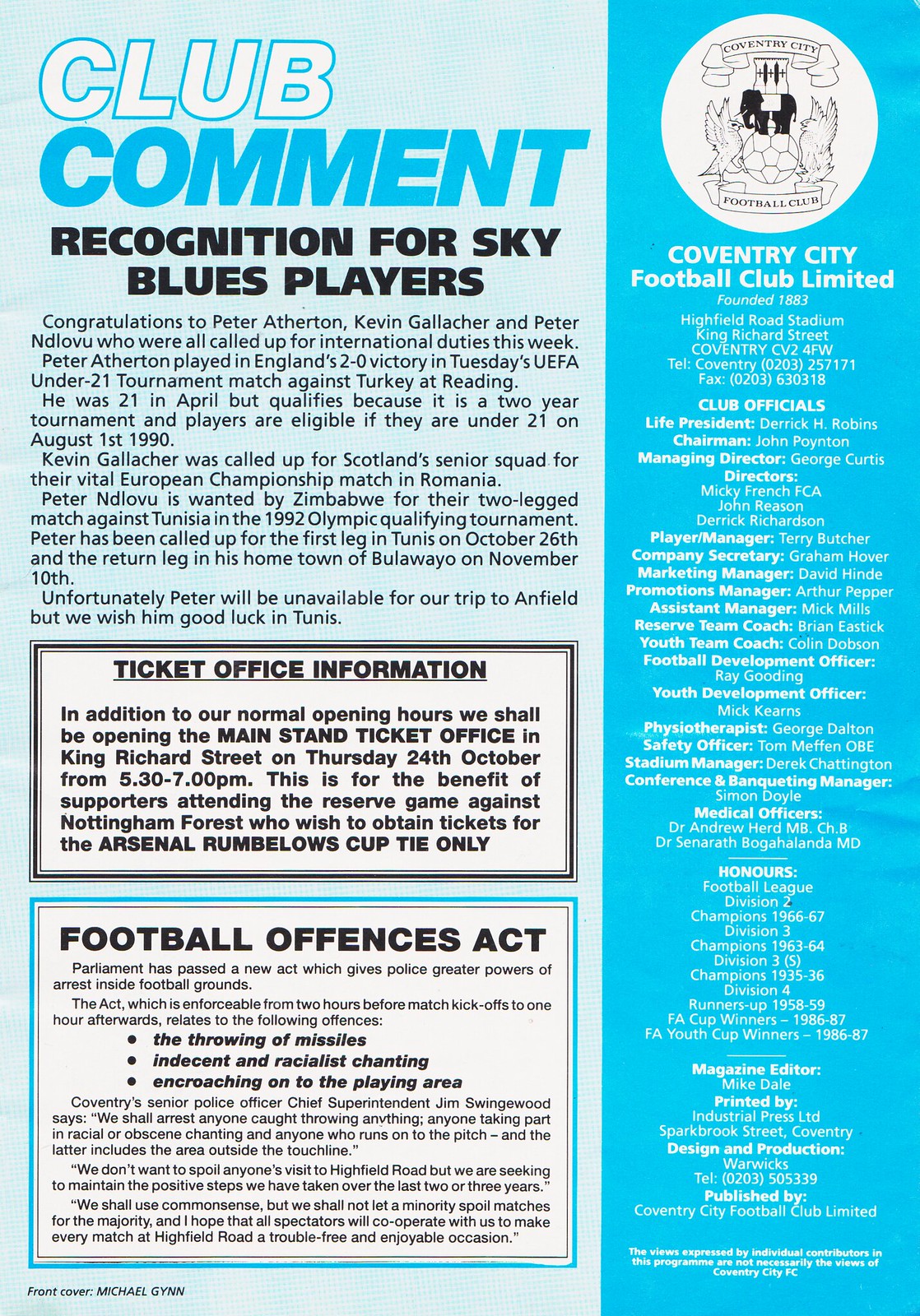The image is an announcement flyer for a sporting event organized by the Coventry City Football Club in England. The flyer, which features a background of light blue and teal blue hues, is split into two sections: about two-thirds of it on the left side has a lighter blue background, while the remaining one-third on the right side has a slightly darker blue but still light background.

At the top of the flyer, prominently displayed in bold, italicized, and sans-serif fonts, is the title "Club Comment," with "Club" in white letters outlined in blue and "Comment" in blue text. Below this header, in non-italicized, black sans-serif font, it reads "Recognition for Sky Blues Players," congratulating Peter Athron and another player named Kevin.

Additionally, there are sections with essential information, including a ticket office notice enclosed in a white rectangle with a black border, and details about the "Football Offenses Act" outlined in a blue and thin black inner border. On the left side, a circular icon representing the Coventry City Football Club is displayed, along with official club information in white text. The information includes warnings for attendees about appropriate behavior, such as not throwing objects, engaging in racist behavior, or invading the pitch. The flyer also lists the club directors, hours, and editors for their magazines.

Overall, the flyer appears to be the last page of a program, emphasizing the event's rules and recognizing key players, set against a detailed and visually segmented blue-toned background.